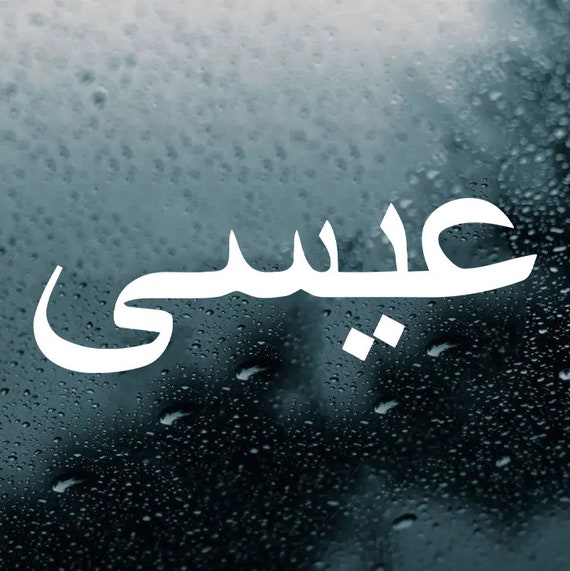The image depicts a rain-splattered window, resembling a windshield on a rainy night, with raindrops scattered across the glass. The background transitions from a dark, rain-spotted lower right corner to a lighter, off-white upper left. This gradient effect creates a moody, almost melancholic atmosphere. Across the center of the image, in elegant white calligraphy, is text in what appears to be Arabic. The script, featuring intricate swoops and two diamond-shaped dots beneath it, stands out against the dark and gradually lightening background. The text is ornate and decorative, stretching horizontally across the middle of the image, and is contrasted beautifully by the blue undertones of the raindrop-streaked glass behind it.